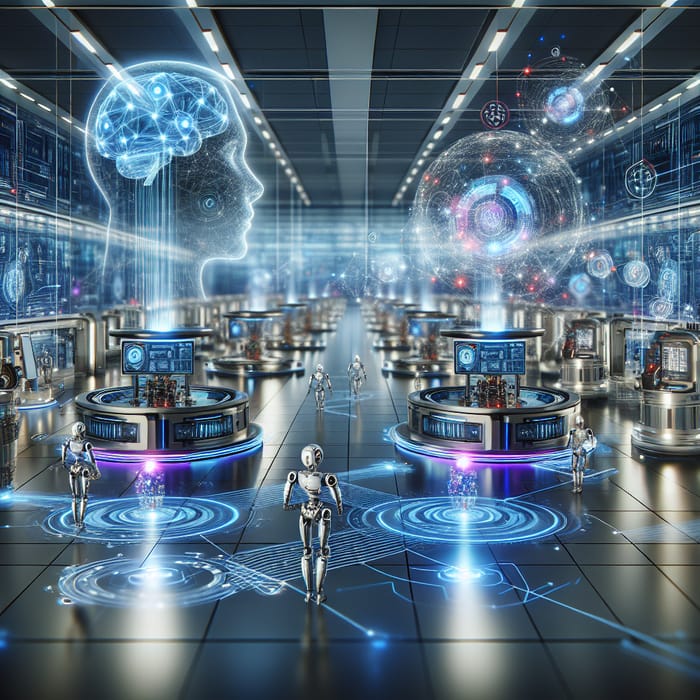The image showcases a highly futuristic, digital drawing dominated by robots and a hub of advanced technology. Central to the composition is a prominent robot positioned at the bottom center, surrounded by five other human-like robots dispersed across a tiled floor that reflects gray light. Blue crop circles and intricate lines are projected onto the floor, accentuating a sense of technology and motion. Floating circular stations, resembling nodes in the New York Stock Exchange, extend down the center of the image with each station featuring round, flat-screen terminals displaying identical images. Above, holographic projections animate the scene; the top left corner displays a side profile of a human face with a brain mapped out with targets, highlighting different points of focus. The right-hand section of the ceiling features additional round images, reminiscent of planets or celestial objects. The color palette is predominantly blues and grays interspersed with subtle purple hues, contributing to the abstract, otherworldly ambiance of the scene.